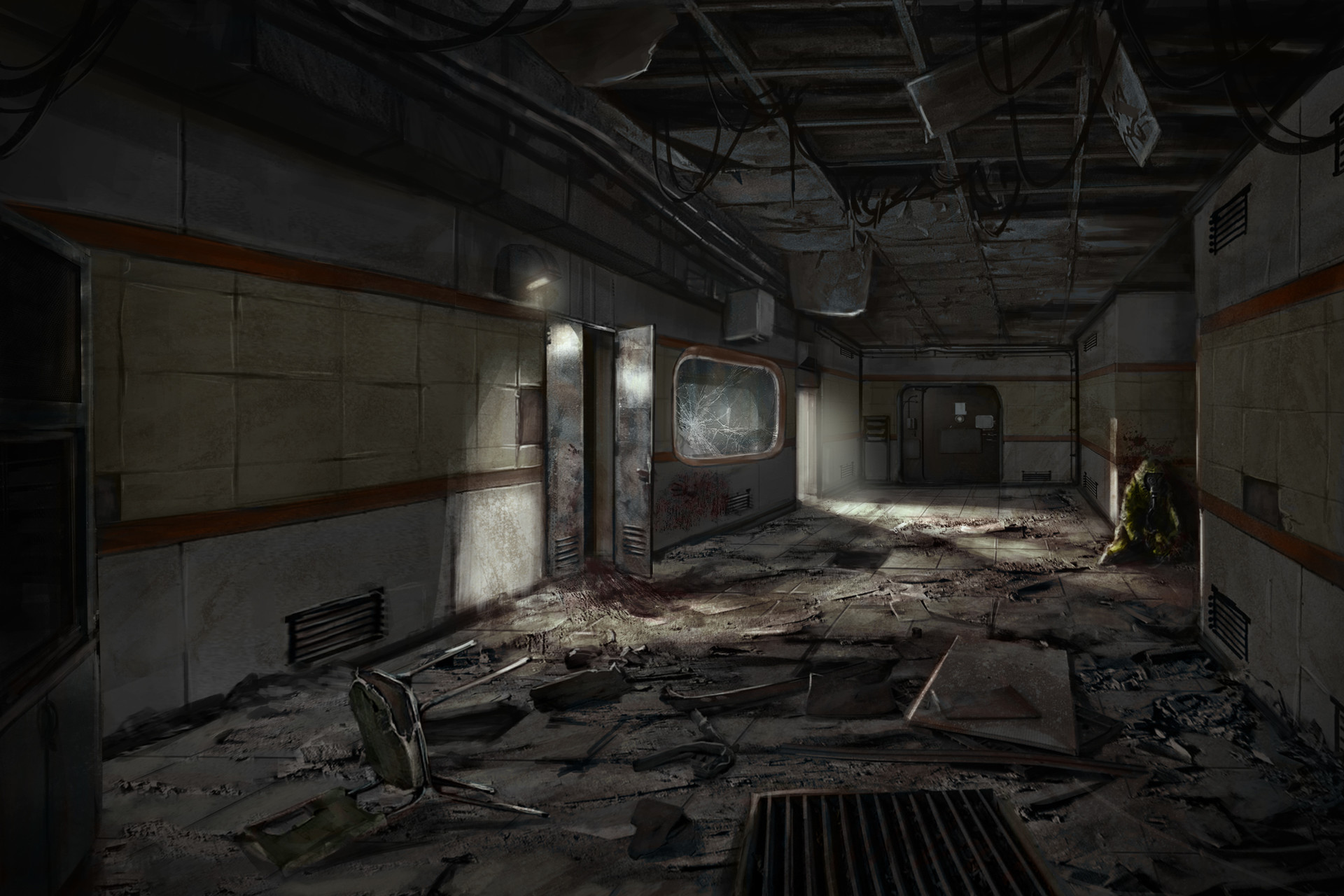The image depicts a screenshot from a stylized video game, possibly Dead Space, set in an abandoned research facility that resembles an old factory or medical ward from the 1950s. The room is in ruins, characterized by broken items, shabby and ripped-apart floors and ceilings, and broken panels on the walls. A window, which looks like a viewing window next to two lockers, adds to the eerie setting. The floor is covered in dust and dirt, with stools lying scattered and ceiling boards hanging precariously. A white, dingy appearance envelops the facility, with walls that have degraded over time.

In the scene, a person in a yellow hazmat suit is crouching and leaning against the wall on the right side of the image, amidst the carnage of what appears to have been a significant earlier conflict. Additionally, there is a vent grate and an open door on the left from which light streams in, casting a whitish glow across the center and left of the room. Despite this light source, the room remains predominantly dark, adding to the overall atmosphere of abandonment and desolation.